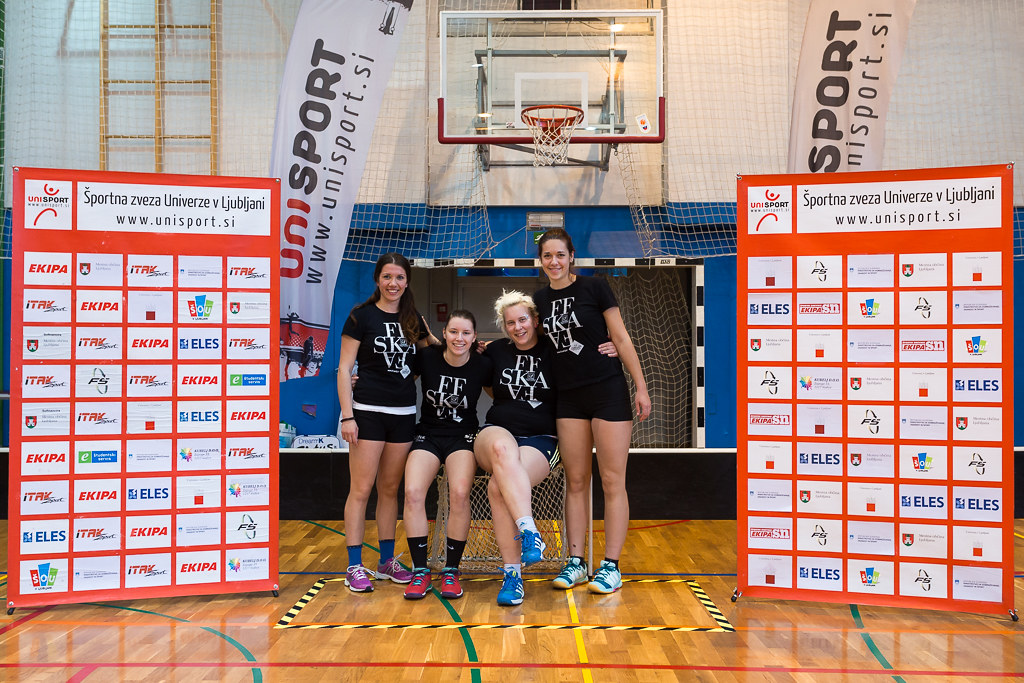The photograph captures four young female athletes posing in a gymnasium, positioned beneath a basketball hoop. The women are dressed uniformly in black athletic tops with white lettering, black shorts, and sneakers of varying colors. Two athletes are standing at the far left and right, tenderly grasping the shoulders of the two seated in the middle, who are hugging around their waists. They are all smiling.

The backdrop features red sponsor banners that flank both sides of the group, each covered with white logos and text. The banners prominently display the phrase "Sportna Zvezda Univerze V Ljubljani" along with the website "www.unisport.si". Additionally, above the group, white banners with the same text and website hang, further indicating their affiliation with Unisport. The wooden gym floor and the overall setting suggest this photograph was taken in an Eastern European athletic facility.